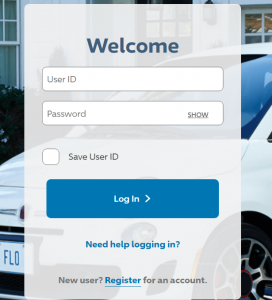The image is a screenshot with a photograph as the background, showcasing the front driver's side of a white vehicle parked near a white building. Superimposed on this background is a semi-transparent grey vertical rectangle, allowing partial visibility of the photograph on both the left and right sides.

At the top center of the grey rectangle, approximately four lines down, there is a bolded, large blue text that reads "Welcome". Beneath this heading lies a white rectangle outlined in grey, serving as a text input field labeled "User ID" in grey text on the left-hand side. Below this, there is a second, identical white input box, labeled "Password" in grey on the left side. Within this password box, on the right side, the word "SHOW" is displayed in grey, all caps, and underlined.

Further down, approximately four lines below the password box, is a white check box outlined in light grey. To the right of this check box is a black text reading "Save User ID". Positioned a couple of lines below this is a blue rectangular login button, which contains the text "Log In" in white, accompanied by a right-pointing arrow resembling a sideways "V".

About three lines beneath the login button, centered in blue text, is the phrase "Need help logging in?", followed by an additional prompt roughly four lines down that reads "New User?" in grey, centered in black text. The word "Register" follows, displayed in blue, underlined, and then "for an account" in grey text.